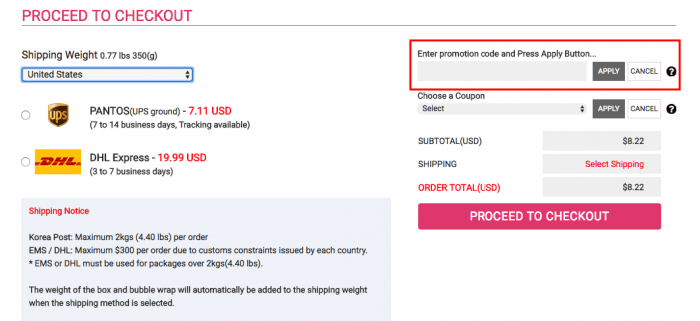In the top left corner of the image, red text indicates a shipping weight of 0.77 pounds (350 grams). Encased within a blue border, the information specifies the United States as the destination. Below, several shipping options are detailed: 

- UPS Ground is not selected and shows a cost of minus $7.11 USD, with an estimated delivery time of 7 to 14 business days and tracking available.
- DHL Express, highlighted in red letters, costs $19.90 USD, with a delivery window of 3 to 7 business days.
- Korea Post can handle a maximum of 2 kilograms (4.4 pounds) per order.
- EMS is mentioned as needing to comply with a $300 maximum per order due to customs controls from various countries.
- Packages over 2 kilograms (4.4 pounds) must use either EMS or DHL.

The weight of packaging materials such as the box and bubble wrap is automatically added to the shipping weight upon selecting the shipping method.

In the top right corner, a red border prompts users to enter a promotion code and click the 'Apply' button. Below that, a red bar allows users to choose a coupon, and includes ‘Apply’ and ‘Cancel’ options. The order summary shows a subtotal of $822 USD in gray, which also reflects the shipping selection. The overall order total is displayed as $822 USD in total. A prominent red rectangle at the bottom of the image guides users to 'Proceed to Checkout.'